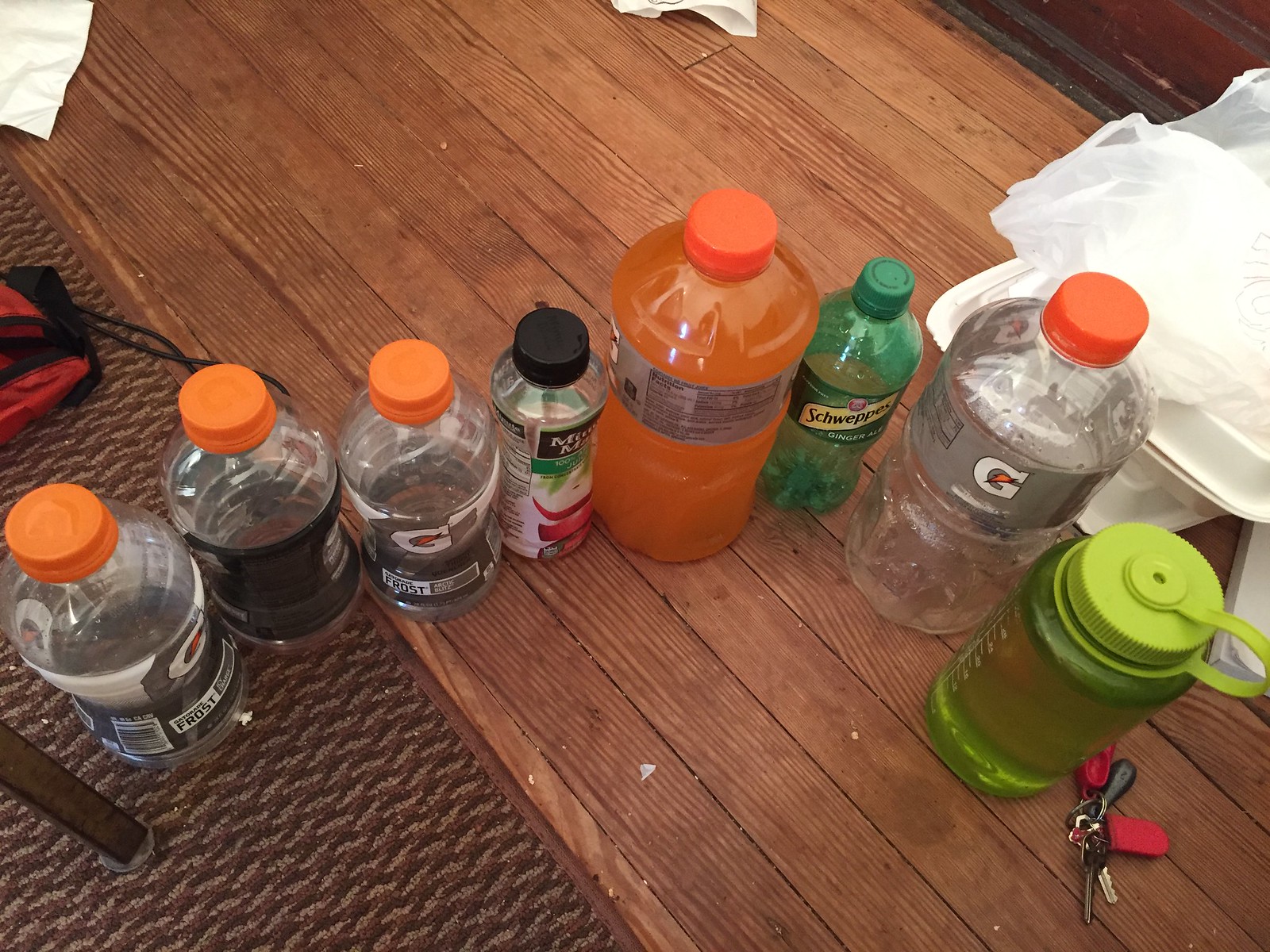The photograph depicts a slightly curved row of eight bottles, standing on a brown hardwood floor that transitions into a brown carpet featuring a tan and brown squiggly pattern. The line-up begins on the left side with three empty Gatorade bottles, each with orange caps. Adjacent to them, there's an empty Minute Maid apple juice bottle with a black cap. Next in line is a full orange Gatorade bottle. Following this, there is an empty Schweppes ginger ale bottle, distinctive due to its green color and green cap. Further along, another empty Gatorade bottle with an orange cap is seen. The row concludes with a large green reusable water bottle that has measurement markings on its side, capped with a solid lime green top. To the right of the bottles, a set of keys with red and black keychains are placed on the floor, accompanied by stacked white takeaway trays and a white shopping bag. In the background to the left, a part of a rug, a chair leg, and a red and black bag are partially visible.